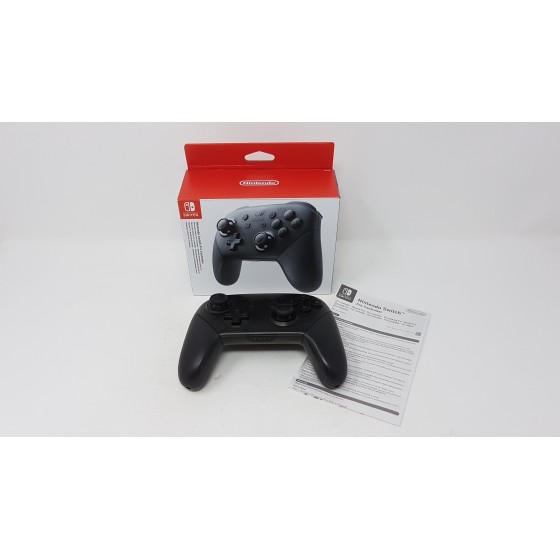The picture features a Nintendo Switch Pro Controller against a white background. The centerpiece is the black controller itself, which has a typical rectangular body with two protruding handles creating an upside-down U shape. On the right side, it's flanked by a white instruction manual with black lettering that's too small to read. Behind the controller is its packaging box, predominantly white with red accents, including a top section with a white circle containing the word "Nintendo" in white letters inside an oval. The front panel of the box showcases a detailed black image of the controller, highlighting its buttons, including the dual joysticks and the D-pad, more clearly than the actual controller. The box also has a punch-out for retail display, suggesting it was designed for a store shelf.